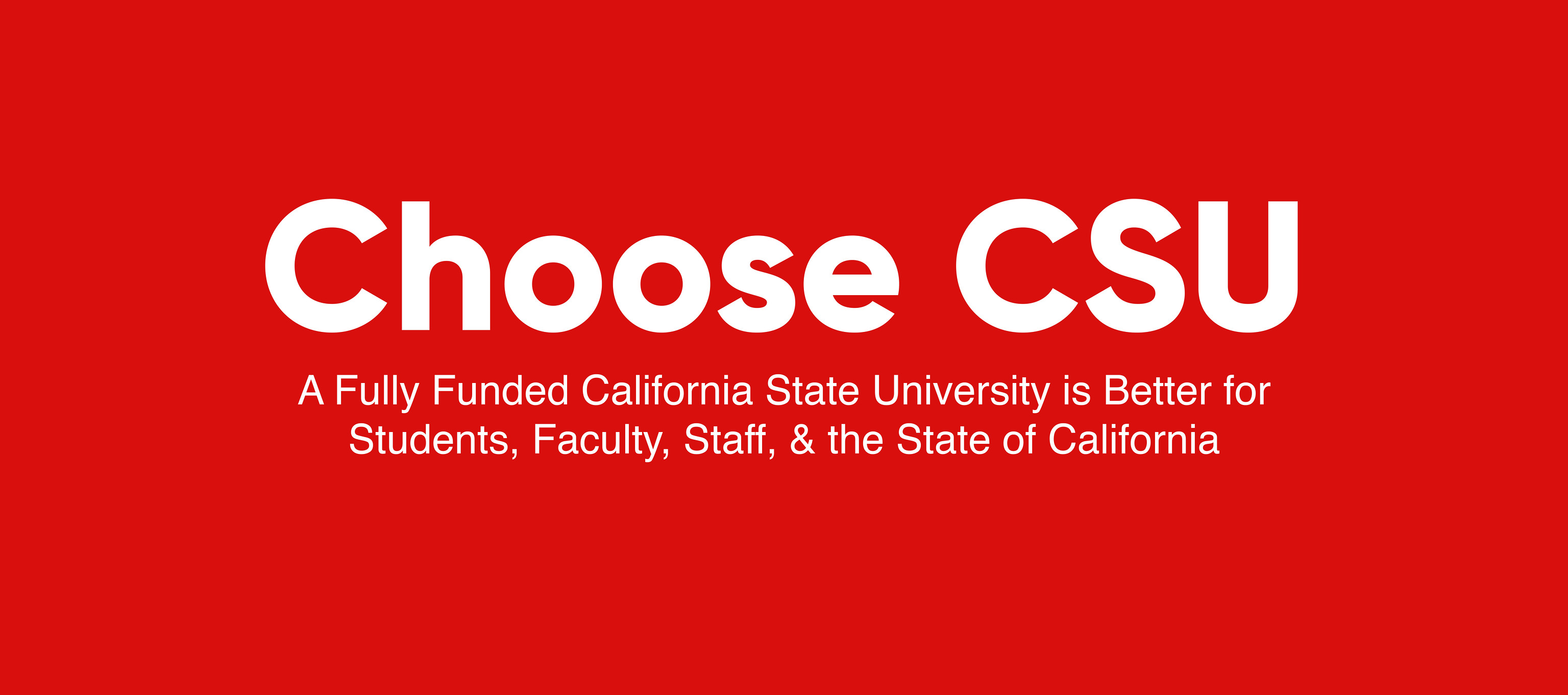The image is a horizontal advertisement banner with a bright red background. The banner is strikingly simple, featuring centered white text. The large, bold white print at the top reads "CHOOSE CSU." Below that, in smaller white letters, it states, "A FULLY FUNDED CALIFORNIA STATE UNIVERSITY IS BETTER FOR STUDENTS, FACULTY, STAFF, & THE STATE OF CALIFORNIA." The entire text is aligned both horizontally and vertically in the center, and no additional information, such as websites or credits, is present on the banner.